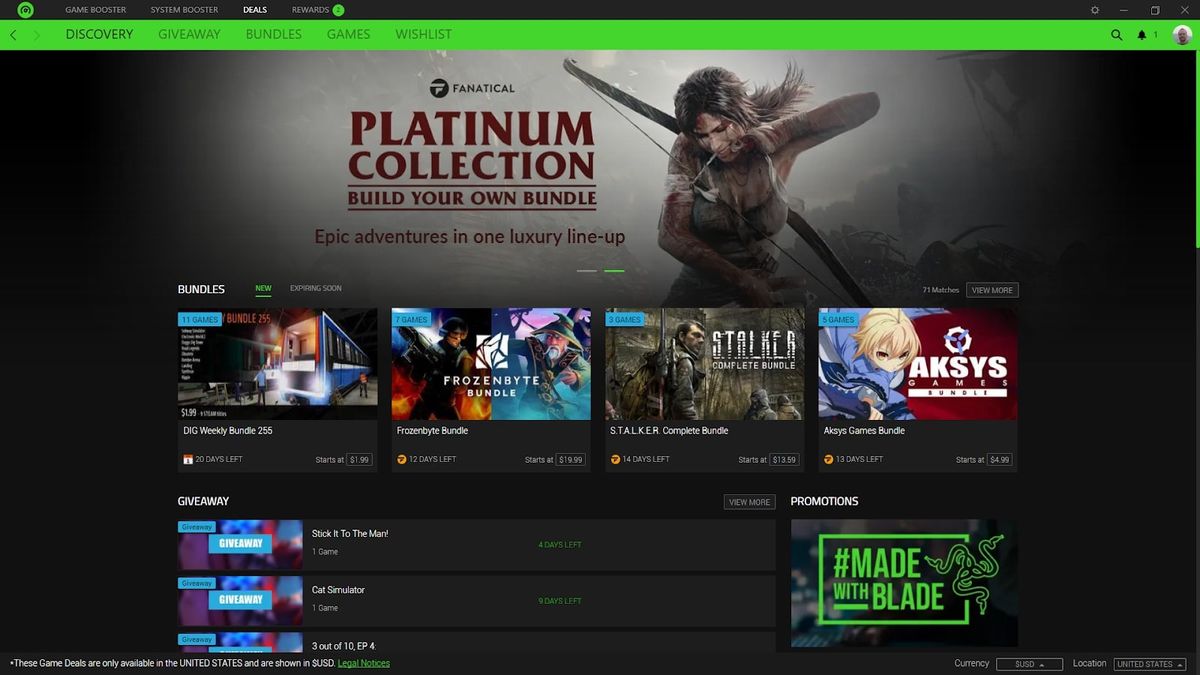This screenshot captures a web interface with an organized layout and various interactive elements. The top section features a black header with a small green circle containing a logo on the left, followed by a horizontal list of navigation options: "Game Booster," "System Booster," "Deals" (highlighted in a brighter white), and "Rewards." Adjacent to these, a green circle is also visible. On the far right, there are icons for settings, minimizing, and closing the window.

Directly beneath this, a vivid lime green banner displays further navigation options: "Discovery," "Giveaway," "Bundles," "Games," and "Wishlist." To the banner's right, there are icons for search (magnifying glass), notifications (bell), more options (three dots), and a user profile picture.

The central content area has a gray background flanked by black margins. Prominently, the word "Fanatical" is displayed, followed by a title "Platinum Collection" and a subheading "Build Your Own Bundle, Epic Adventures in One Luxury Lineup" in burgundy text. The image features a graphic of a woman wielding a bow and arrow. Below, a white capitalized text reads "BUNDLES," with "NEW" in green text and "expiring soon" in smaller letters. Further down, the interface lists various bundle options, including "DIG Weekly Bundle 255," "Frozen Byte Bundle," "Stalker Complete Bundle," "Axis Bundle," "Axis Games Bundle," all under the designation "Made with Blade Promotions."